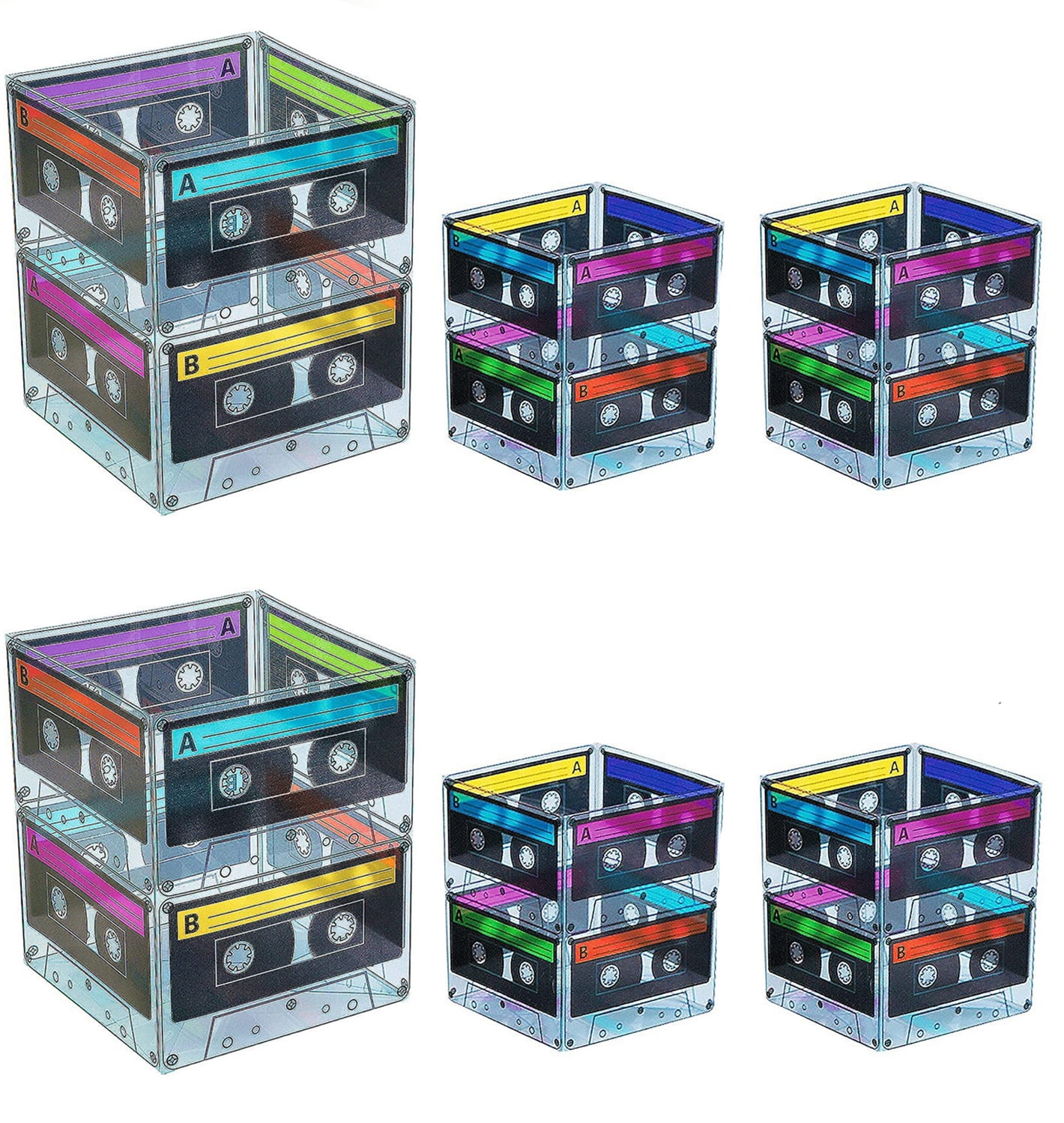Against a plain white background, the image features six intricately handcrafted boxes arranged in two rows of three. Each row is oriented such that the left front corner of the boxes is closer to the center, creating an angled perspective. These boxes, appearing to be made from clear plastic or acrylic, each replicate the design of black cassette tapes, complete with reels visible through their transparent sides.

The drawn cassettes boast colorful banners with horizontal lines and capital letters 'A' or 'B' on them. Notably, the first box in each row is the largest, measuring about an inch and a half in both height and width, while the remaining boxes are slightly smaller, approximately an inch in both dimensions. Each cassette box alternates its letter such that on one side, 'A' is on top with 'B' on the bottom, and on the reverse, 'B' is on top with 'A' at the bottom. The vibrant banners come in hues of purple, green, blue, yellow, and red, adding a distinct pop of color to the otherwise minimalist design.

This intricate and detailed arrangement creates an impression of cassette tapes being cleverly repurposed into functional storage boxes.